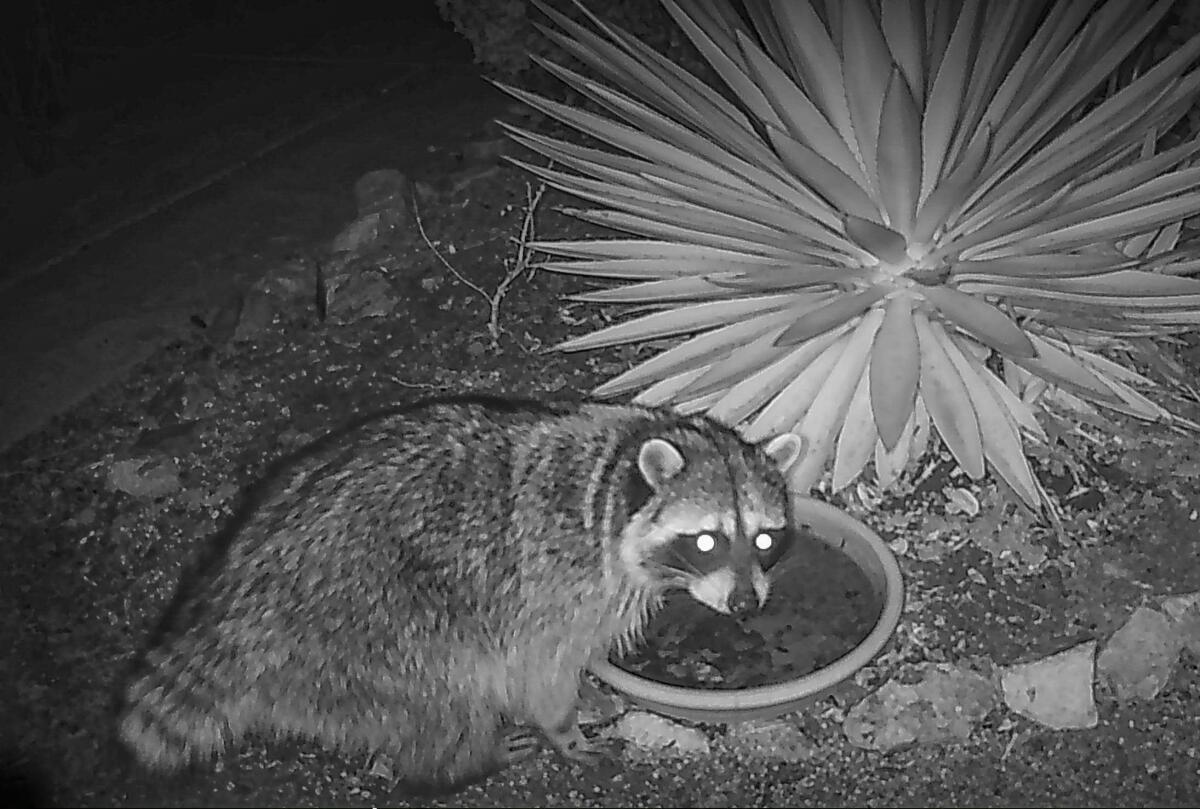This black and white photographic image appears to be captured using night vision technology, likely from a security camera setup outdoors. The scene centers on a large, furry raccoon with distinctive black rings around its eyes, which are reflecting brightly from the camera flash. The raccoon is positioned in the middle of the photograph, with its tail towards the bottom left corner and its head turned to gaze directly at the camera, suggestive of an alert and curious expression.

The raccoon seems to be investigating or consuming something from a shallow dish or bowl, probably containing food or water, placed next to a lush plant with radiating leaves. This plant is rooted within a small garden plot, meticulously bordered by a circle of arranged rocks. The foreground is composed of soil and scattered stones, whereas the top left part of the image fades into darkness, emphasizing the nocturnal ambiance of the scene. The photograph is devoid of any text, compelling viewers to focus purely on the stark interplay of light and shadows highlighting this nocturnal encounter.